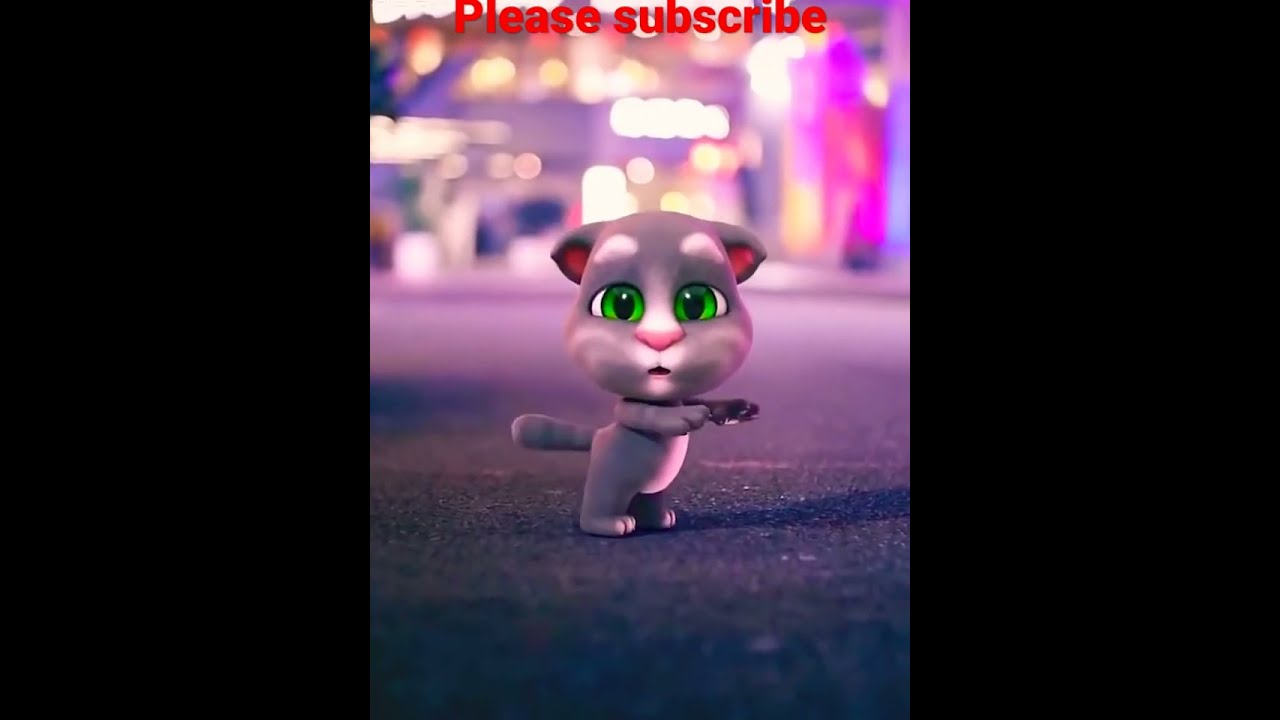The image is a computer-generated artwork depicting a cartoon-like gray cat with an exaggeratedly oversized head and a tiny body. The cat, standing on its hind legs, has a distressed or surprised expression characterized by vivid green eyes, white eyebrows, and downcast ears with pinkish interiors. Its arms are extended in front of it, and it sports a club-like tail. The cat's fur is predominantly gray with a lighter gray on its belly and white tips on its toes. The background features an out-of-focus series of city lights, creating a blurred, colorful urban backdrop. The cat appears to be standing on an asphalt street, and text at the top of the image reads "please subscribe" in red lettering. There are also two vertical black bars on either side of the image that are about three and a half inches wide and four inches tall, though their purpose is unclear.